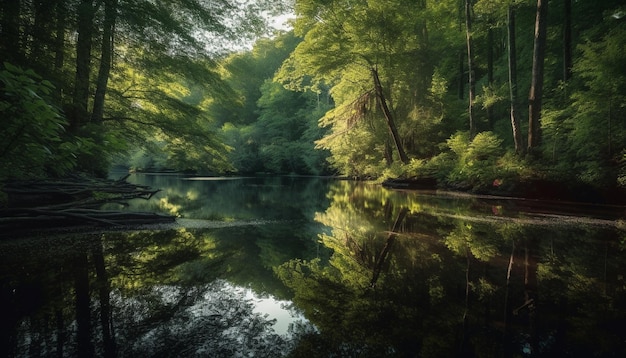A mesmerizing landscape image captures an ethereal lakeside scene nestled in the heart of a dense forest. Deciduous trees with soft, almost blurry branches frame the composition, casting varied hues of sap green, viridian, and olive across the tranquil water. The scene hints at a sunny day, though the light filters softly from behind the trees on the left, leaving portions of the photograph, particularly the bottom right and top right, in shadowed darkness. The serene water, devoid of movement, mirrors the sky and scattered limbs, while dappled sunlight and floating pollen speckle its surface. There's a sense of mystique and calm, accentuated by subtle colors – greens, yellows, light browns, black, and a distant red plant whose reflection shimmers on the right side of the image. The overall atmosphere is both peaceful and enchanting, inviting viewers to lose themselves in the harmony of nature's hidden corner.